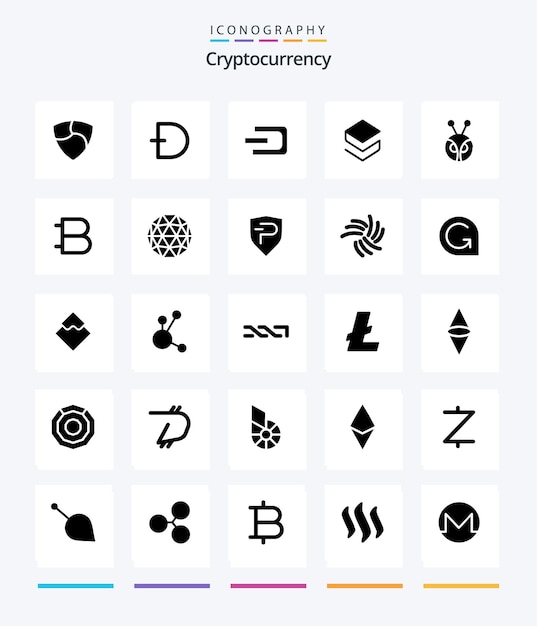This is a detailed image of a poster dedicated to the iconography of cryptocurrency designs. At the top of the poster, the word "Iconography" is prominently displayed in black sans-serif font, with the word "Cryptocurrency" underneath. Below the title, there are five colorful dashed lines in a rainbow gradient, featuring shades of turquoise, purple, pink, orange, and yellow. 

The main body of the poster features 25 distinct cryptocurrency icons, arranged in a 5x5 grid on a white backdrop with each icon displayed in a small white square. These icons are all rendered in black, presenting a variety of digital and monetary symbols. The first icon in the top-left corner resembles a shield, followed by an icon of the letter 'D' with a dash through the middle. Other icons include one that looks like a mirrored 'E,' which resembles a computer power sign, and icons with letter 'Bs' and various other structures and symbols.

At the bottom of the image, similar colorful dashed lines in light blue, purple, maroon, orange, and yellow are neatly aligned, mirroring the decorative accents at the top. The entire poster maintains a primarily black-and-white color scheme with the colored dashes serving as vibrant decorative elements.